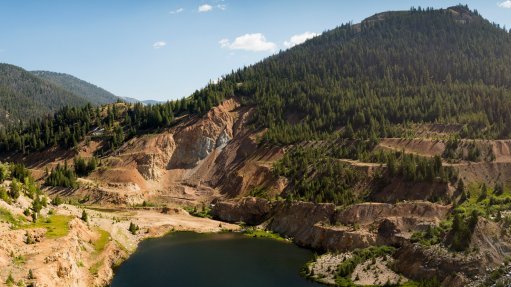This image portrays a picturesque mountainous landscape dominated by a large, brown mountain covered in lush, dark green trees. The mountain features stepped formations, which could be either natural terraces or remnants of man-made construction, complete with some cave-like entrances. A path meanders along the left side of the mountain. A prominent shadow stretches over the scene, likely cast from another peak behind the photographer.

In the foreground, there is a blend of light brown dirt and lighter green grass, interspersed with small trees and scrubs. Beige-colored cliffs, possibly sandstone, frame a body of water, suggesting a lake or river nestled within the rugged terrain. 

In the background, more hills and distant mountains emerge, filling the landscape. The sky overhead is a vibrant blue, dotted with a few white clouds, enhancing the natural beauty of the scene. This setting, reminiscent of the American West or similarly arid regions, captures the raw and diverse elements of nature in a single frame.